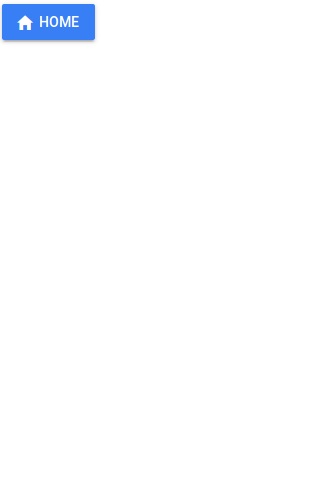A small blue rectangle, approximately three inches wide and two inches tall, serves as the focal point of this image. The background within the rectangle is a medium blue color. Positioned on the left side of the rectangle is a simplistic white house icon, featuring a triangular roof and a vertically oriented rectangle representing the door. To the right of this icon, the word "HOME" is displayed in bold, white, uppercase letters. The overall design is clean and minimalistic, with no additional elements present in the image.